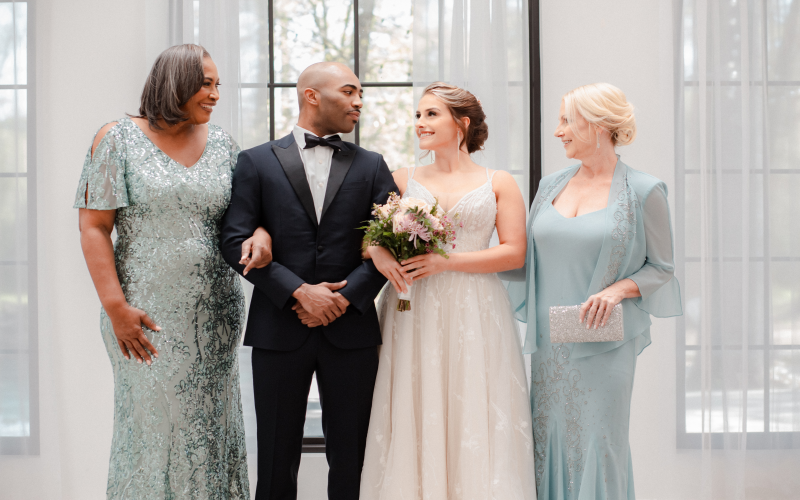This detailed wedding photo captures four elegantly dressed individuals posing together. At the center are the bride and groom, their arms interlocked and smiling warmly at each other. The groom, an African-American man with a bald head, wears a classic black and white tuxedo with a black bow tie. The bride, a white woman, dons a stunning white dress and holds a bouquet of pink flowers with green leaves. Her long hair is styled in an elaborate updo.

To the groom's left stands an African-American woman, possibly his mother, sporting a silvery brocade gown with cold shoulders and short hair styled in a bob. On the bride's right is an older Caucasian woman, likely her mother, who has short blonde hair and wears a light blue dress with a delicate gauzy sleeve jacket. She holds a silver pocketbook in her left hand.

The background of the photo features three large windows draped with silky white curtains that allow a hint of the greenery outside to show through. The setting is elegant and serene, with a color palette of green, blue, white, black, and pink enhancing the celebratory atmosphere.